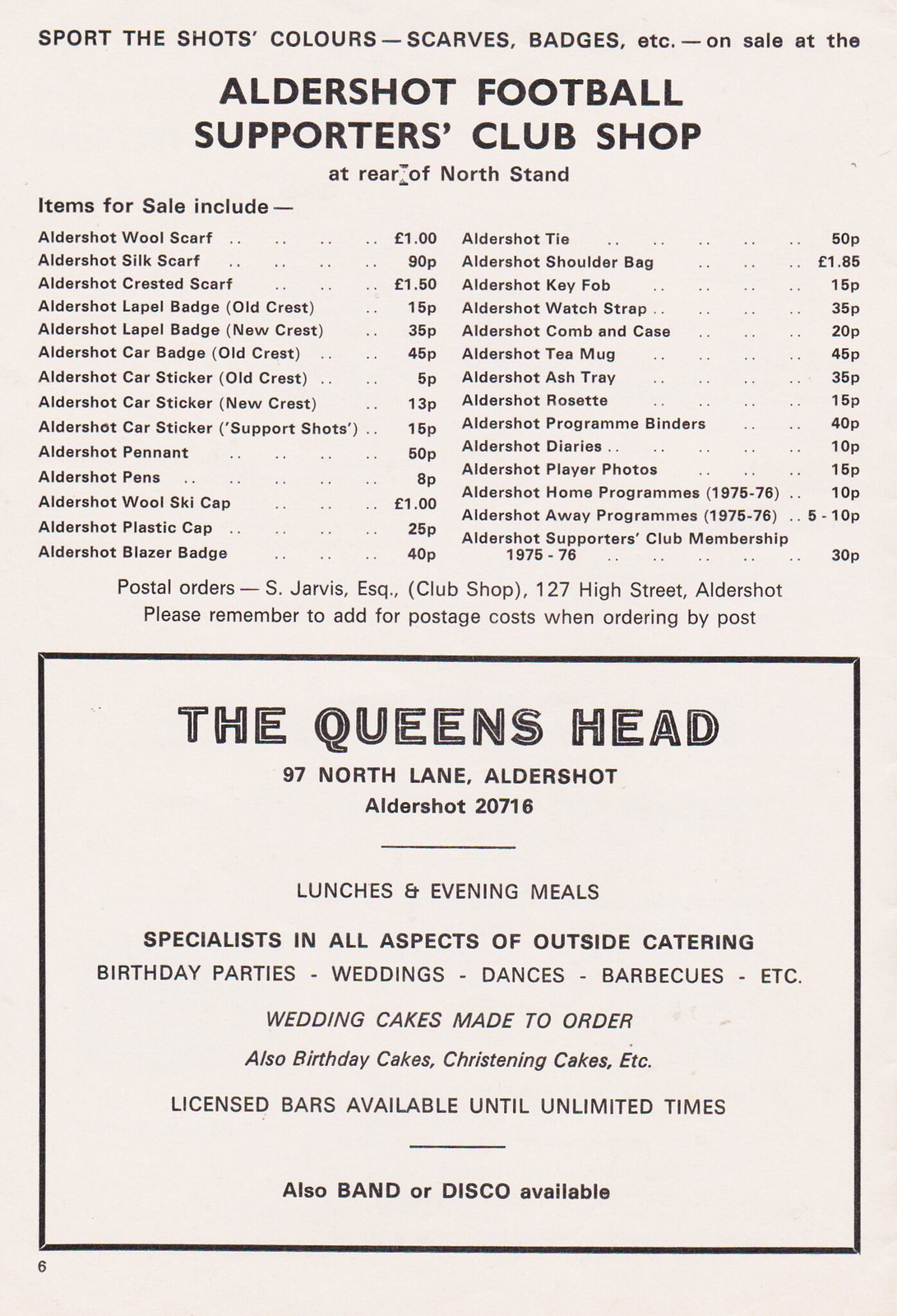The image appears to be an old, vertically aligned rectangular advertisement, possibly from a newspaper or magazine page, promoting the Aldershot Football Supporters Club Shop. At the top, bold, all-caps black text states, "ALDERSHOT FOOTBALL SUPPORTERS CLUB SHOP." Beneath this title, smaller black text reads, "Support the Shots. Colors, Dash, Scarves, Badges, Etc. On sale at the Aldershot Football Supporters Club Shop at the rear of North Stand."

The advertisement features two columns detailing merchandise available for purchase, each item starting with "Aldershot." The list includes:

- Wool Scarf, one pound
- Silk Scarf, ninety pence
- Crested Scarf, one pound fifty pence
- Lapel Badge (Old Crest), fifteen pence
- Car Badge, price not specified
- Car Sticker, price not specified
- Pennant, price not specified
- Pens, price not specified
- Wool Ski Caps, price not specified
- Plastic Caps, price not specified
- Blazer Badge, price not specified
- Tie, price not specified
- Shoulder Bag, price not specified

Adjacent to this merchandise list, it notes that postal orders are available from 127 High Street, Aldershot, with a reminder to include postage costs when ordering by mail.

At the bottom of the advertisement, a large bordered section promotes "THE QUEEN'S HEAD." The address is given as 97 North Lane, Aldershot, with the phone number Aldershot 20716. It elaborates on the food and services offered, including:

- Lunches and evening meals
- Outside catering for events such as birthday parties, weddings, dances, barbecues, with licensed bars available until unlimited times
- Wedding cakes, birthday cakes, and christening cakes made to order
- Availability of bands or disco services for events

Overall, the advertisement gives a nostalgic look into the offerings and services of the Aldershot football supporters community and their sponsors.